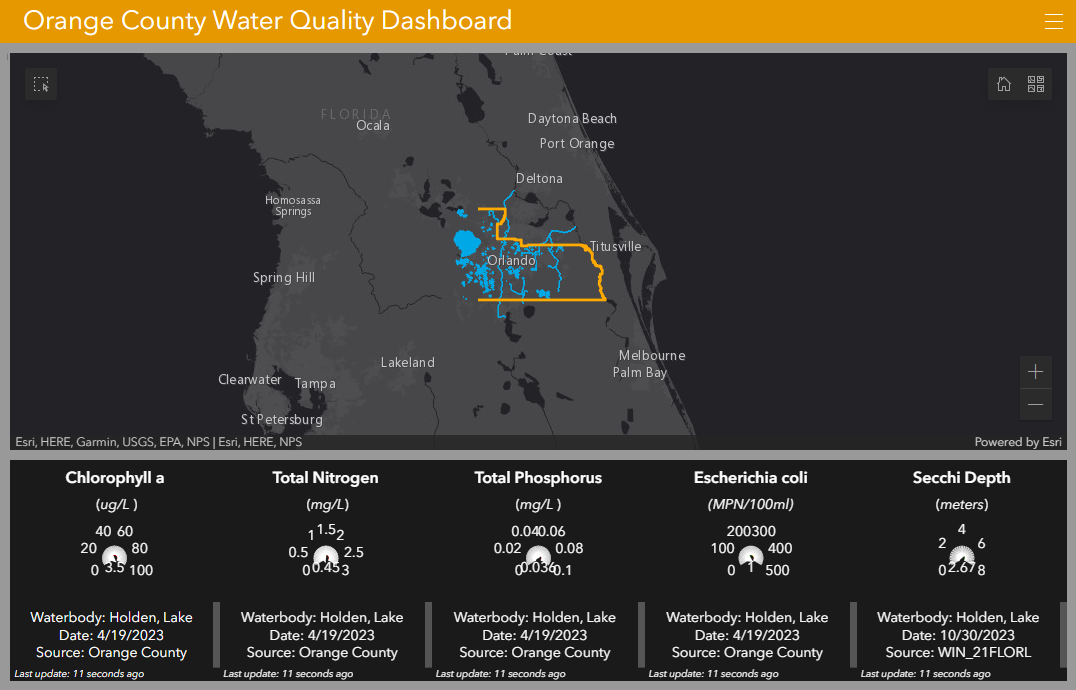This image is a screenshot taken from a website in landscape mode. Across the upper left corner, there is an orange strip featuring the title "Orange County Water Quality Dashboard." The content is divided into two main sections. The top section displays a map of Orange County with the highlighted areas in orange, likely representing water quality data specific to Orange County. The surrounding blue areas, encompassing the city of Orlando, appear to indicate bodies of water such as lakes and rivers where water quality is being monitored.

In the bottom left corner, there is detailed information about Holden Lake's water quality metrics dated April 19th, 2023. The chlorophyll level is listed at 3.5, although the acceptable level for chlorophyll isn't provided. Total nitrogen is measured at 0.45, and total phosphorus at 0.036. The E. coli count is noted as 1, and the Secchi depth, indicating water clarity, is recorded at 2.67 meters. These numbers might be significant to those familiar with water quality standards, suggesting a medium range in some parameters, which could be a point of concern for residents and environmental experts.